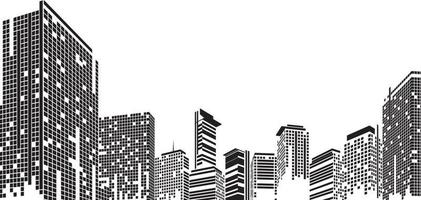This is a detailed black and white digital sketch of a city skyline arranged in a somewhat U-shaped curvature. The composition features 10 buildings of varying heights, starting with the tallest skyscraper on the left, which gradually descends in height towards the center before rising again on the right. The buildings are meticulously detailed, showcasing a blend of architectural designs with square-shaped windows predominantly filled in black to suggest a nighttime scene, though a few windows are left white, possibly indicating illuminated rooms. The background of the image is stark white, accentuating the intricate contrasts and details of the buildings. Some structures include horizontal lines running through them, adding additional texture to the sketch. The overall perspective appears as if one is looking upward at the skyline, emphasizing the towering nature of the edges.